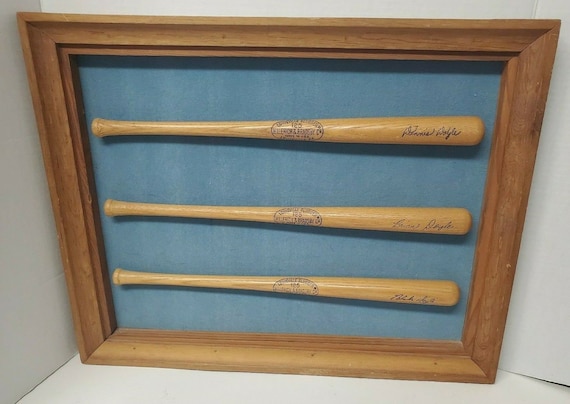The image showcases three wooden baseball bats encased in a light brown, unstained wooden frame. The frame, predominantly filling the view, has a distinctive design with an outer edge protruding towards the viewer and an inner edge recessed, creating depth. Each bat, light brown in color, is mounted against a bluish backing. The bats are slightly angled, with the handle grips on the left and the bat heads on the right. The top bat appears marginally larger than the bottom bat, possibly due to perspective. All three bats bear cursive signatures towards the right ends, though the names are not fully legible, with the surname "David" discernible on the second bat. At the center of each bat, there is a prominent black stamp featuring a circular text encircling a symbol. This assembly is set against a white backdrop, with a glimpse of a white surface below, possibly in a corner of a gray or light-colored room, giving off a professional, perhaps homemade display vibe.